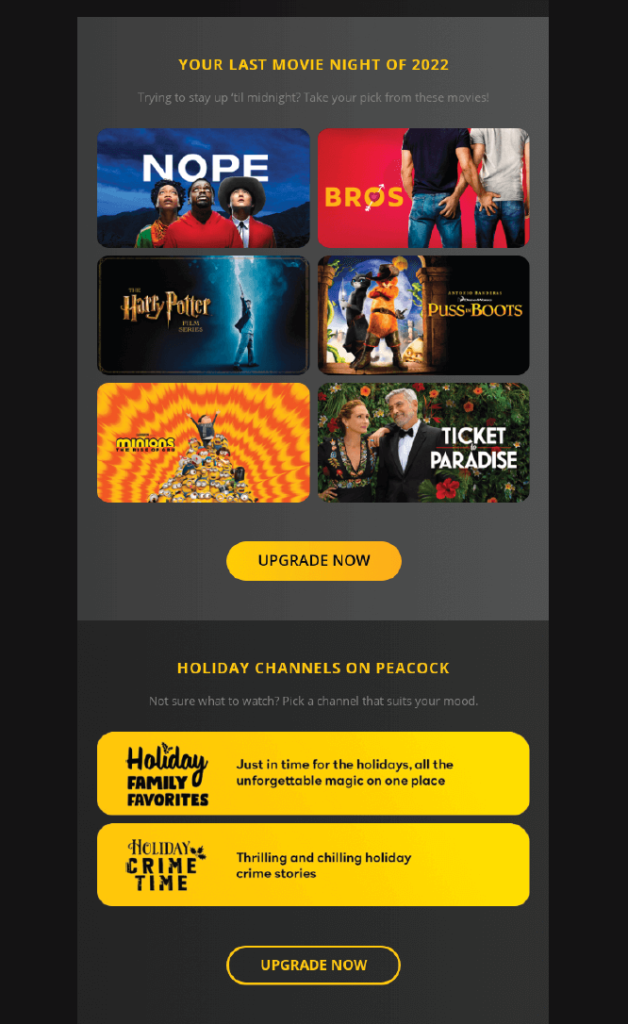This is a detailed screenshot of a movie or streaming service interface. The backdrop is black, providing a stark contrast to the large, vertical, dark gray box dominating the center of the screen, extending from the top to the very bottom of the display. At the top of this gray box, centrally positioned, the text reads "Your Last Movie Night of 2022," suggesting a curated selection for the year's final movie night.

Six movie thumbnails are showcased within the gray box, arranged in two columns with three on the left and three on the right. The featured films include "Nope," "Harry Potter," "Minions," "Bros," "Puss in Boots," and "Ticket to Paradise." These selections hint at a varied mix of genres and audience appeal.

Beneath the thumbnails, a prominent yellow button displays the call-to-action text "Upgrade Now," indicating a prompt for users to enhance their subscription or viewing experience. Further down, the interface highlights specific holiday-themed viewing options, with the header "Holiday Channels on Peacock" in bold letters.

Two yellow rectangular buttons follow, labeled "Holiday Family Favorites" and "Holiday Crime Time," likely leading to collections of holiday films categorized by genre. At the very bottom of the screenshot, another yellow "Upgrade Now" button is partially visible, suggesting the image might be slightly cropped at the bottom edge, as the content seems to extend below the visible portion of the screen. The top portion of the gray box does not align precisely with the top of the black background, enhancing the impression that the image capture is incomplete.